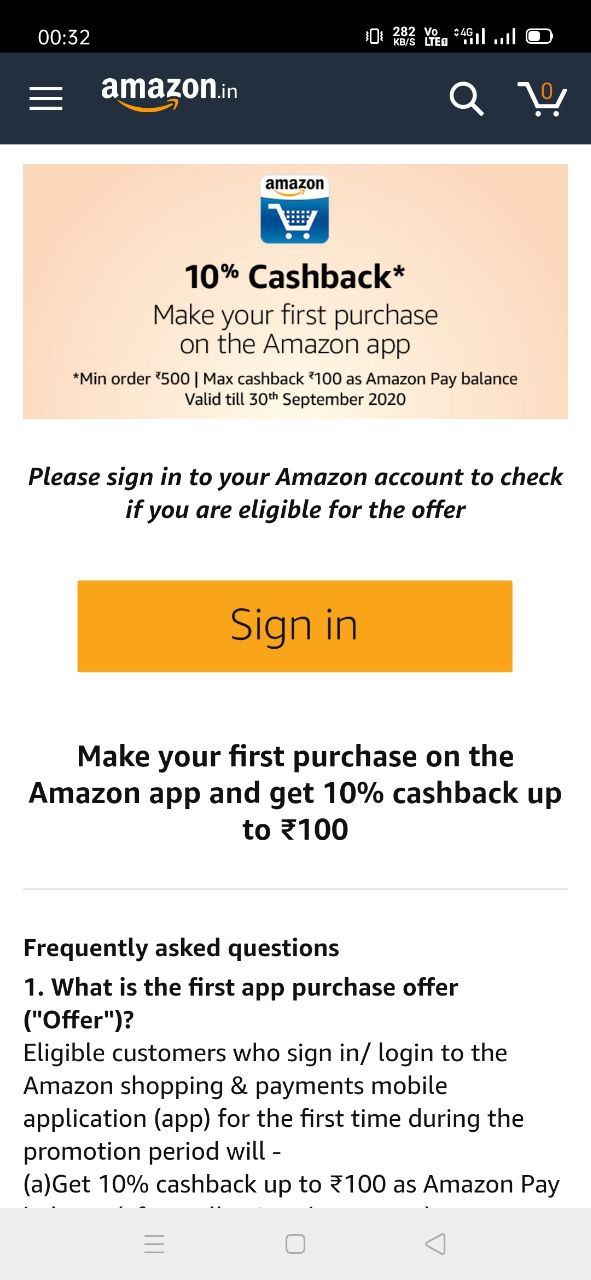In this image, a smartphone screen displays the Amazon app interface. At the top of the screen, a dark navy blue or black banner shows the time "00:32" in white font on the upper left corner. On the upper right corner, six icons, including the battery and Wi-Fi indicators, are visible.

Just below this banner is the Amazon header. On the far left, three parallel lines represent the menu options. To their right is the Amazon logo. On the far right, there are two additional icons: a white magnifying glass and a white shopping cart, currently showing zero items.

Below the header, a beige notification box is prominently displayed. It features the Amazon logo and a white and blue shopping cart icon in the middle. There is a message stating "10% cash back on your first purchase on the Amazon app." Beneath this, black text reads, "Please sign into your Amazon account or check if you are eligible for the offer." An orange button with black text labeled "Sign In" appears below this message.

Further down, additional black text advises, "Make your first purchase on the Amazon app and get 10% cash back up to £100." More detailed information follows in a FAQ section, addressing "What is the first app purchase offer?" and discussing eligibility criteria.

At the bottom of the screen, a gray navigation bar is present. On the left, three parallel lines likely represent additional menu options. In the center is either a square or a circle, and on the right, a triangle points to the left.